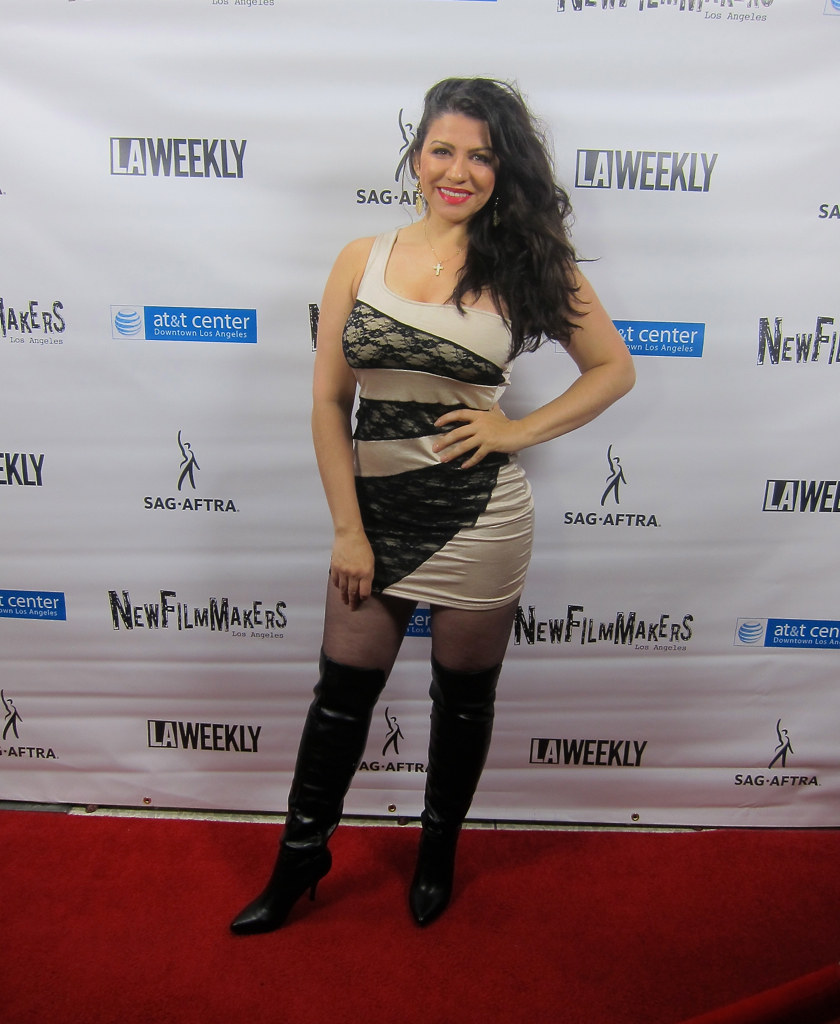This is a detailed photograph of a likely actress at a red carpet event associated with film, evidenced by the backdrop banners displaying logos such as LA Weekly, AT&T Center, SAG-AFTRA, and New Filmmakers. She stands confidently on a red carpet, which is slightly rolled up on the lower right side. The woman is mid-pose, smiling warmly with bright pink lipstick, and has long dark brunette hair cascading elegantly over her left shoulder. She is strikingly dressed in a tight, one-shouldered white dress adorned with black lace detailing across the chest, waist, and forming a triangular pattern down to a miniskirt that ends at her upper thighs. Complementing her outfit, she wears black high-heeled boots that extend above her knees. Adding a touch of glamour, she is accessorized with a cross necklace. Her left hand rests assertively on her hip, her elbow bent, while her right hand hangs down gracefully by her side.